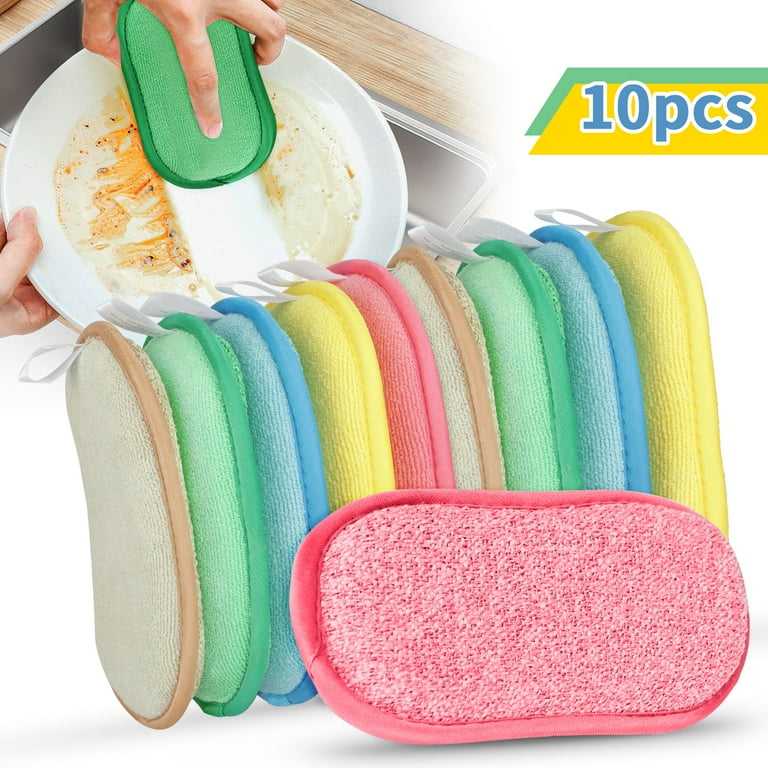The advertisement poster showcases sponges designed for dishwashing. Positioned at the bottom of the image, there’s a neat row of oval-shaped sponges featuring five different colors: beige, green, blue, yellow, and pink, with the sequence repeating. Notably, one pink sponge is placed outside the row on the side. These sponges resemble microfiber shower pads more than traditional rectangular kitchen sponges.

In the background, a partial, close-up photo shows a person cleaning a white plate with leftover food using a green sponge. The plate is held over a kitchen sink. The background of the image is predominantly white. 

At the top right corner of the advertisement, "10 PCS" is boldly written in blue font, surrounded by an overlay of rectangles in yellow and green shapes, signifying that the package contains ten pieces of these multicolored sponges.